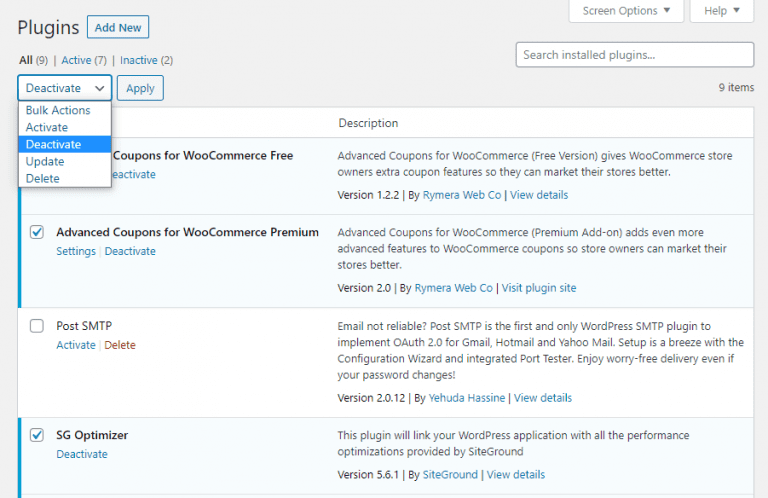In this image, we can see a frozen frame of a computer program's interface, specifically the plug-ins management section. At the top of the interface, there are various options including "Add New," "Deactivate," "Activate," "Update," "Delete," and "Bulk Actions," with an "Apply" button. The captured list of plug-ins includes "Advanced Coupons for WooCommerce Free," "Advanced Coupons for WooCommerce Premium," "Post SMTP," and "SG Optimizer." 

"Advanced Coupons for WooCommerce Free" and "Advanced Coupons for WooCommerce Premium" are both listed, as well as "Post SMTP," which appears to be inactive with options to either activate or delete. "SG Optimizer" is active and it looks like the user intends to deactivate it. On the right side, brief descriptions of each plug-in are provided. At the top, navigation options for "Screen Options," "Help," and "Search Installed Plug-ins" are visible. The list indicates a total of nine plug-ins, with seven active and two inactive, although only the top four are shown in the image.